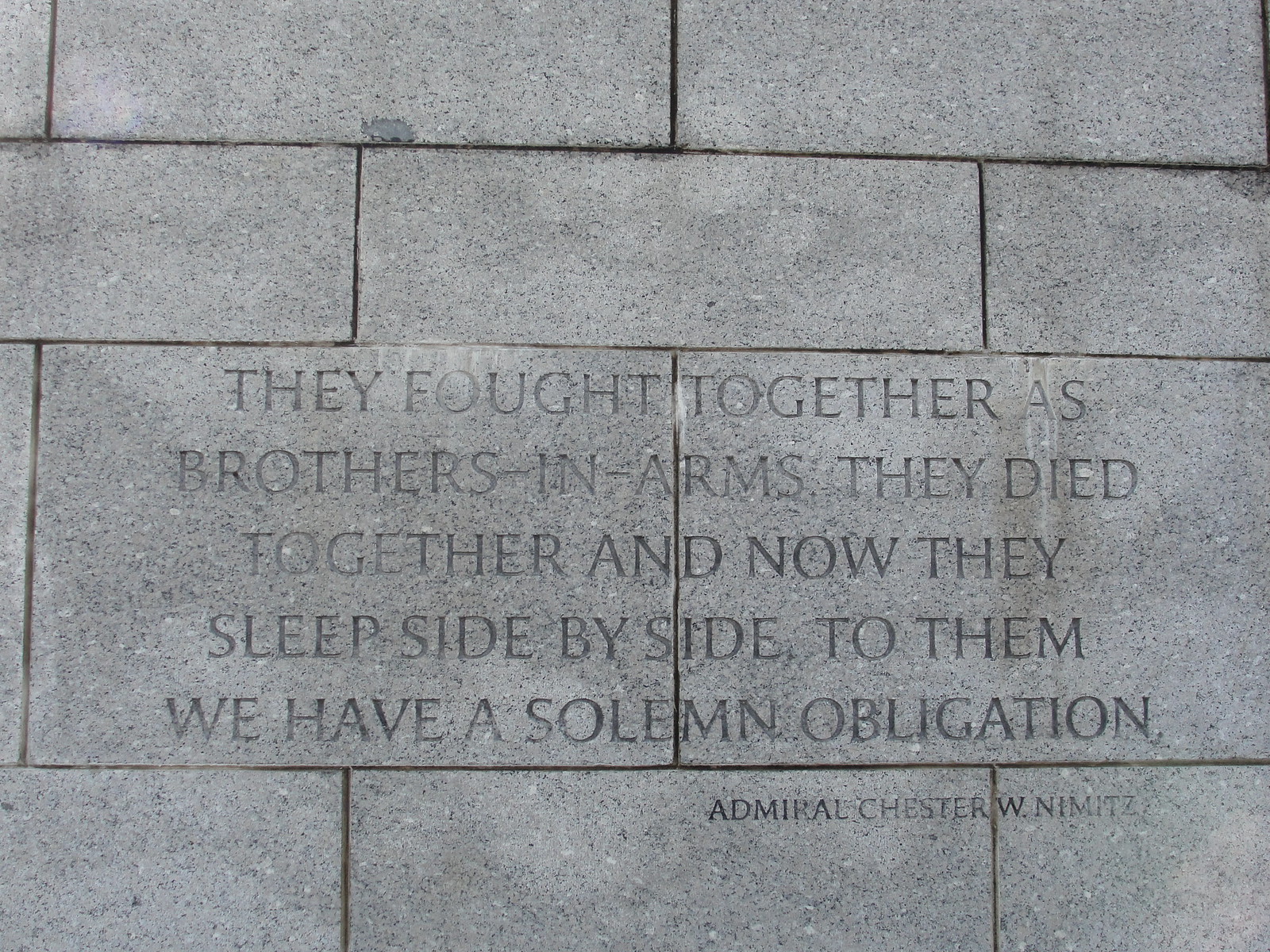The image depicts an engraved gray granite wall, which appears to be part of a larger monument. The engraving, carved into a darker gray section of the wall, reads: "They fought together as brothers in arms. They died together and now they sleep side by side. To them we have a solemn obligation." Beneath this poignant tribute, in smaller all-capital letters, it states, "Admiral Chester W. Nimitz," a notable naval admiral from World War II. The photograph is taken from a slightly diagonal angle, highlighting the subtle shifts in the gray tones of the granite blocks and the inscription. The wall shows some minor cracks, but the inscription remains clearly legible, standing as a somber reminder of the sacrifices made.